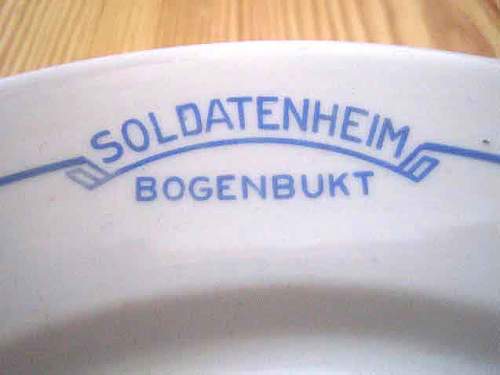This highly detailed close-up image showcases a white ceramic plate on a light wooden table with distinct wood grain lines. The ceramic plate features a prominent blue logo, adorned with the words "Soldatenheim" inscribed in a curved fashion at the top, and "Bogenbucht" directly below. These words are separated by an ornate, curved horizontal divider with intricate detailing. The close-up nature of the photo, covering about 85% of the frame, reveals only a section of the plate, suggesting it could also be a saucer or bowl due to a visible shallow recess. The blue ornamental design runs along the arc of the words, enhancing the aesthetic appeal. Overall, the ceramic detail, coupled with the light wooden backdrop, highlights the craftsmanship and possible origin or brand.